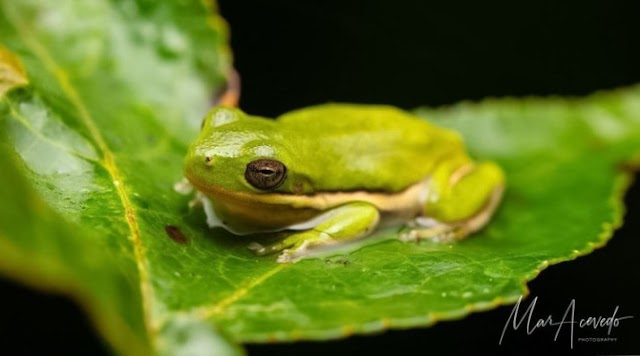This macro shot captures a vibrant green frog with moist, bumpy skin perched on a lush, darker green leaf. The frog has distinct brown eyes, a yellow stripe down its side bordered by a thin brown line, and a white belly. Its spearmint-green body and shiny, slimy texture stand out against the pitch-black background. The frog is facing slightly toward the left, with its head closer to the viewer and its rear receding into the background. The leaf itself is vivid, crisscrossed with light green and yellow veins, accentuated with water droplets. The frog's toes and a faint puddle of liquid beneath it add to the scene's realism. A barely readable, cursive signature is located at the bottom right of the image, possibly reading "Man Alvarado".